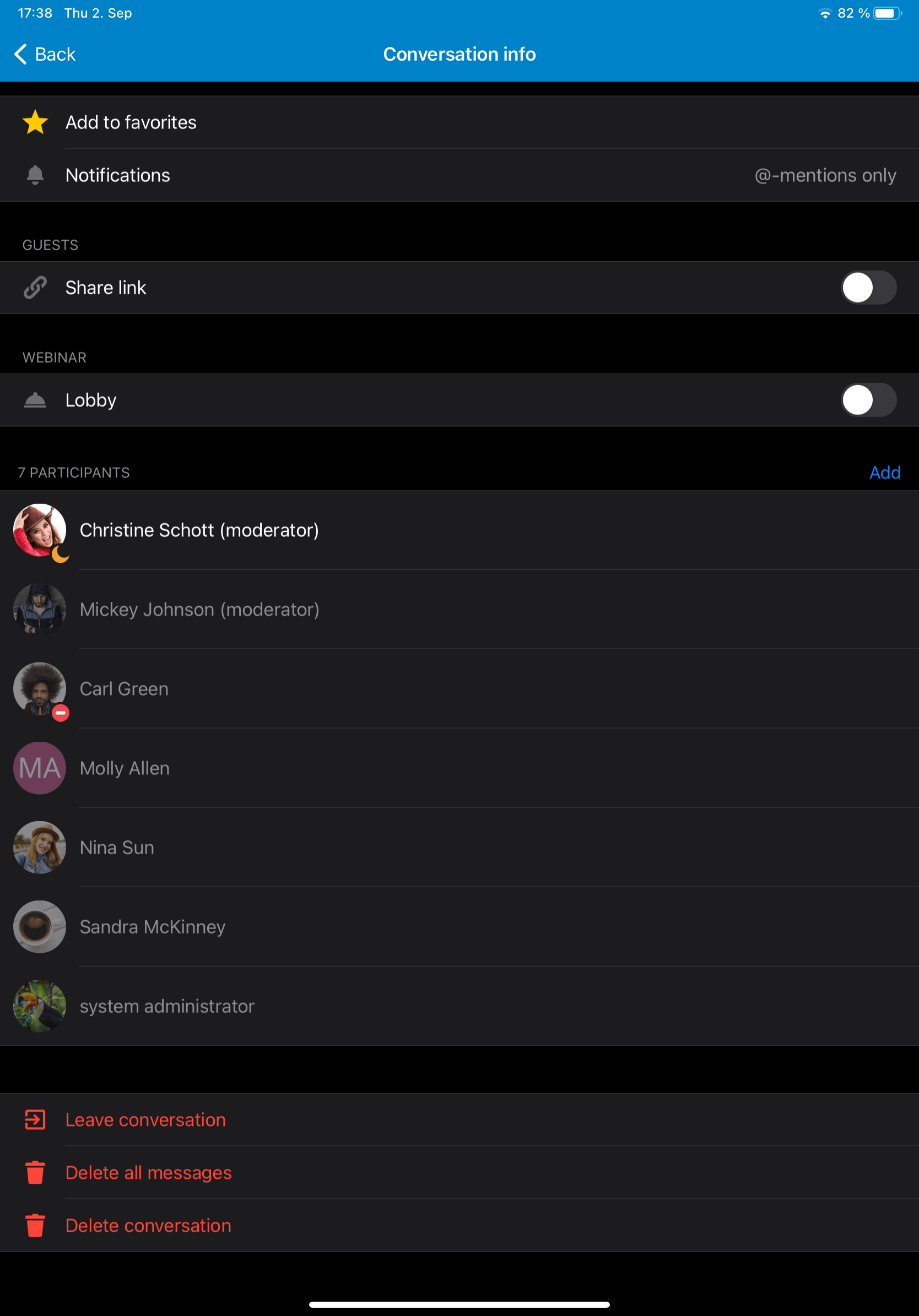A screenshot of a mobile website interface is displayed on a black screen. At the top of the screen, it shows a section titled "Conversation Info." Below this, there are several options listed sequentially: "Add Back," "Add to the List," "Add to Favorites," and "Notifications."

The interface then proceeds to a section labeled "Guests," containing several interactive options and user names. The list begins with "Share Link," followed by "Lobby."

The display then lists several names with their respective roles:
- Christine Schultz (Moderator)
- Mickey Johnson (Moderator)
- Carl Green
- Molly Allen
- Nina
- Nina Sun
- Sandra McKinney
- Susan Ann (Administrator)

Further down, additional options include "Leave Conversations," "Delete All Messages," and "Delete Conversations."